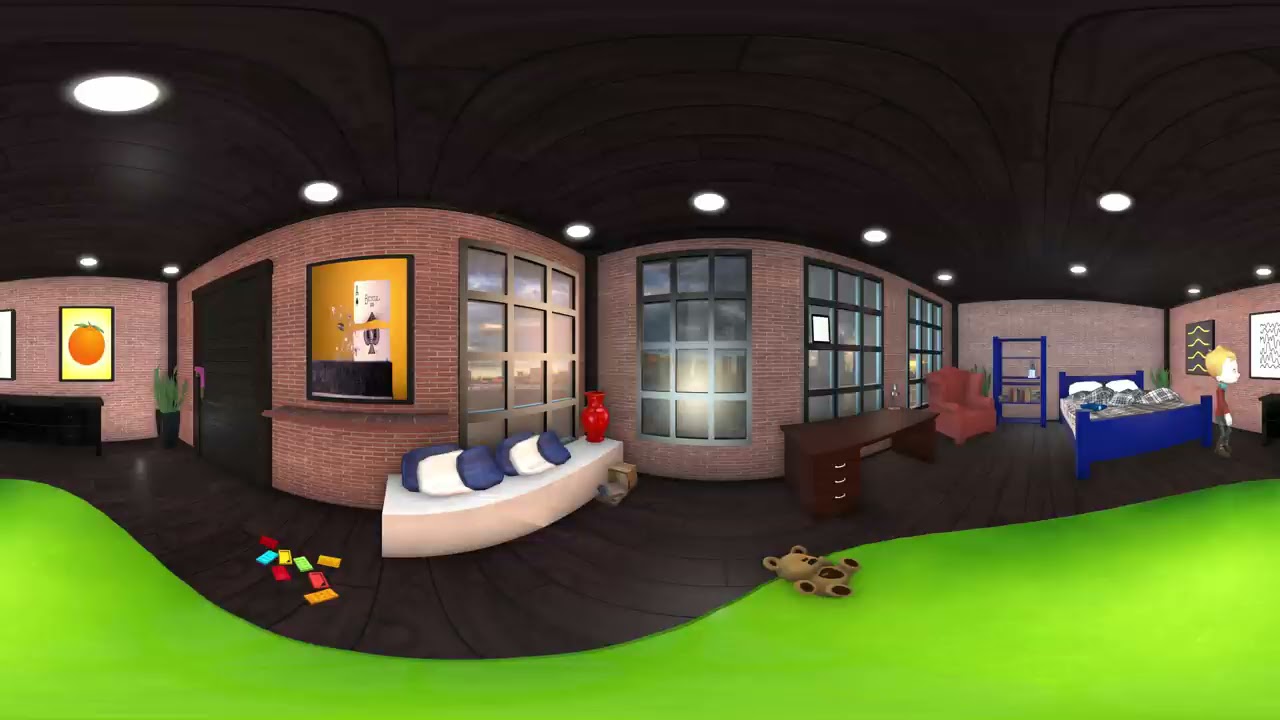The image showcases a meticulously designed furniture store display emulating a cozy, modern bedroom setup. Dominating the forefront is a white sofa adorned with two blue and white pillows, adjacent to which sits a small table with a striking red vase. The scene is set upon a vibrant green curved floor, transitioning into a brown wooden pattern further back. To the right, under a black ceiling punctuated with white circular lights, is a well-arranged bedroom display. This area features a blue bed with plush blankets, a brown chair, and a practical desk, complemented by a small bookcase and several paintings on the walls. Nearby, a stuffed bear and some scattered Legos add a touch of playful realism. The left side of the frame includes a door, a series of pictures, and a prominent poster. The detailed room setup, combined with the presence of an animated little boy character, suggests this is a scene from a computer-generated image designed to resemble a lifelike bedroom.